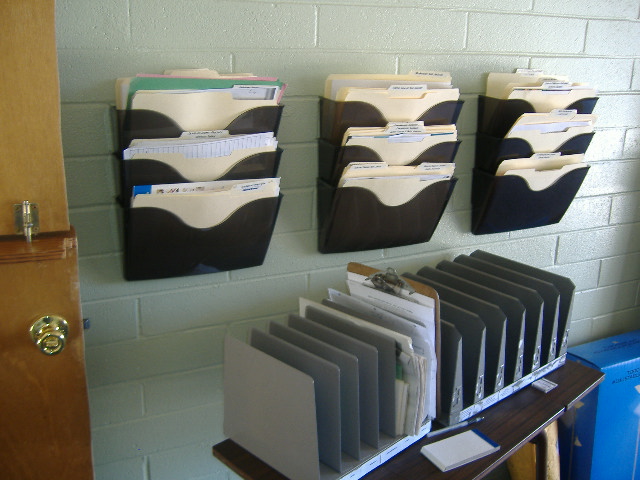In this low-resolution, landscape photograph of an office setting, a white painted brick wall dominates the scene. Mounted on this wall are three black plastic tri-level folders, each designed to accommodate multiple manila file folders, collectively offering storage for 12 distinct areas of files. The files are primarily light beige with one green sheet visible, all neatly organized within their respective compartments. 

Beneath these wall-mounted folders sits a small, dark wooden table. Atop the table are two heavy gray steel file dividers, each capable of holding between five and eight sections. Scattered on the table are a clipboard, a pad of paper, and a pen lying at the edge. 

To the right in the bottom corner of the image, there is a square blue box on the floor. On the left side, an open brown Dutch door with a gold handle and visible lock mechanism separates the top half from the bottom half of the door, highlighting the unique split design characteristic of Dutch doors. Overall, the image conveys a functional office environment meticulously organized for efficient file storage and access.